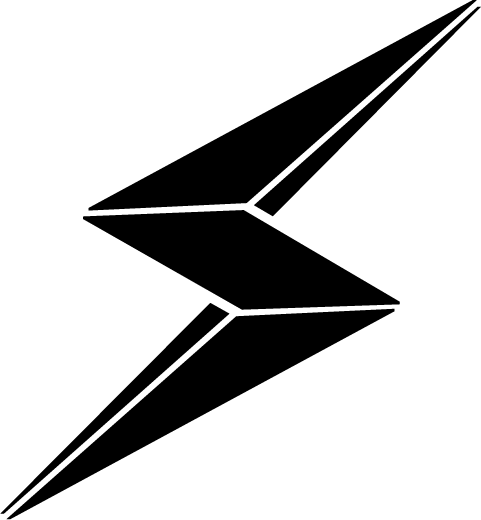The image depicts a minimalist, black and white graphic design resembling a lightning bolt or a sharp, elongated 'S' shape. This symbol is composed of five pointed shapes: four long triangles and a central, elongated quadrilateral (or rhombus) surrounded by white lines creating separation between each segment. The top portion of the lightning bolt points to the upper right, while the bottom extends toward the lower left. The crisp, straight lines and the contrast between black and white lend a striking, modern appearance with a clean, geometric aesthetic.